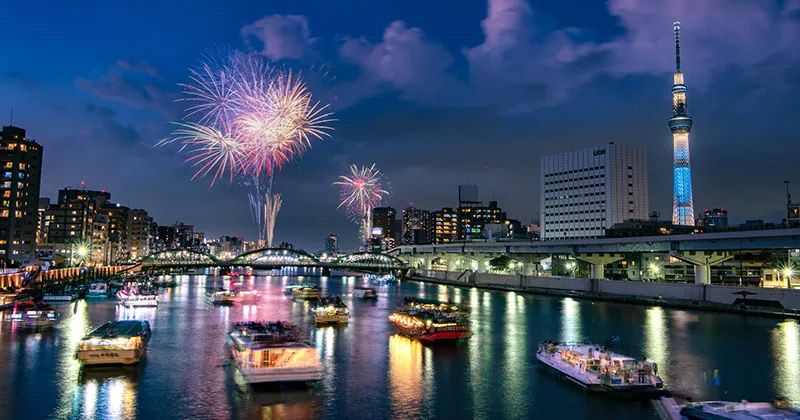The nighttime photograph captures a spectacular scene over a waterfront, featuring a vibrant fireworks display. Brilliant hues of pink, red, cream, and light green light up the dark blue sky, accentuated by beautiful mauve clouds. High-rise buildings, some colorfully lit, stand tall along the horizon, with a prominent needle-topped tower on the right side of the image. The city buildings' lights, along with the fireworks, cast a dazzling array of colors—yellow, green, and blue—onto the relatively still water below. Boats, anchored and illuminated, dot the water's surface, their occupants likely enthralled by the festive fireworks display reminiscent of a major city's 4th of July celebration. The overall scene is both vibrant and serene, with the sky and water reflecting the brilliance of the colorful explosions above.